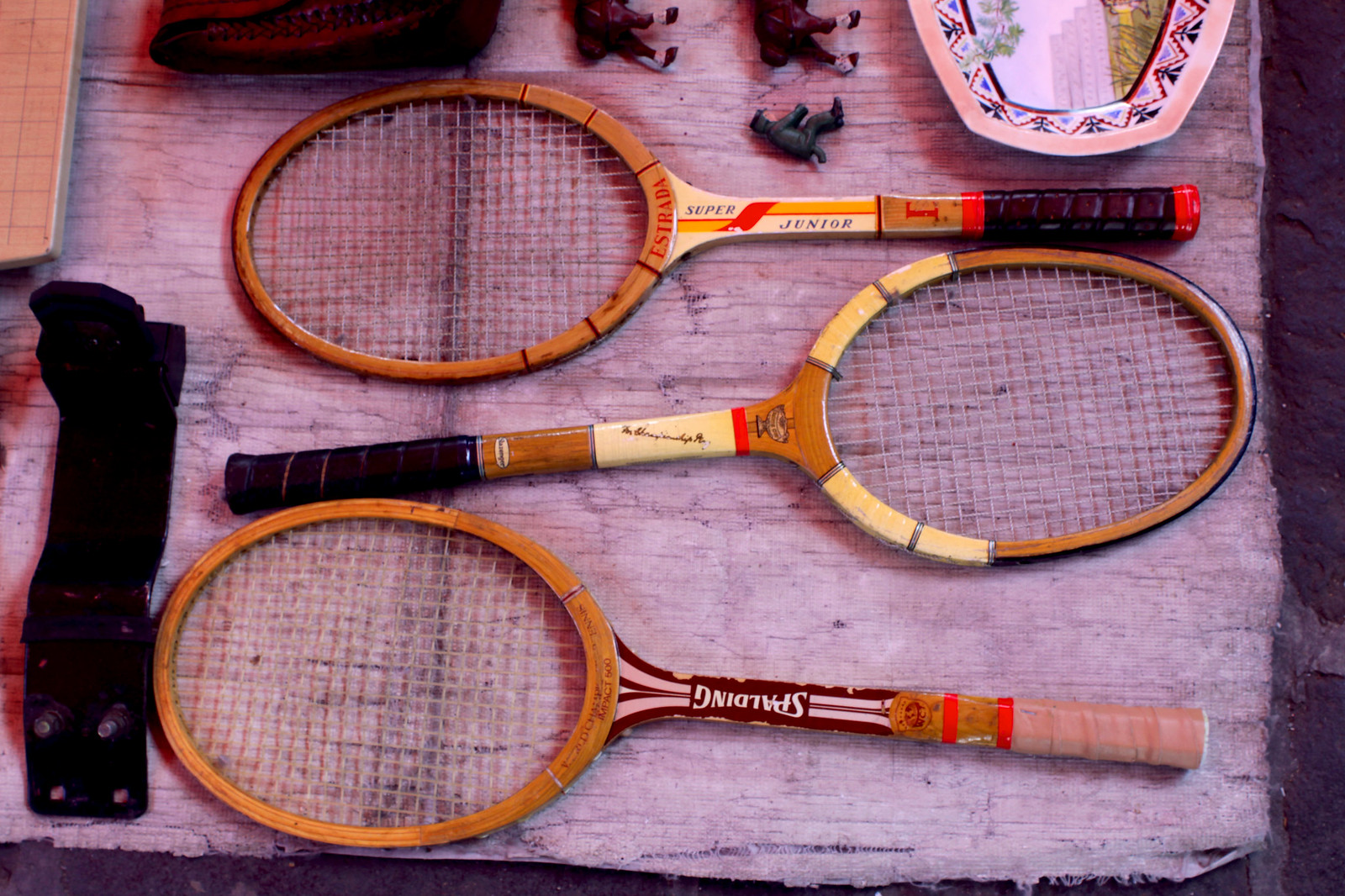This photograph captures an overhead view of a weathered wooden table with a light, almost white appearance, covered in various items suggestive of a garage or yard sale. The main focus in the center are three vintage wooden tennis rackets from what appears to be the 60s or 70s. The topmost racket, marked "Super Junior," is positioned horizontally with its handle wrapped in black tape facing right. Just above it, there is a small black object resembling a toy gorilla. The second racket, situated directly below and oriented in the opposite direction, also features a black-taped handle and has a brown wooden top with yellow edging. The third racket lies beneath them, parallel to the top one, with the word "Spalding" prominently displayed on its handle. The table is notably old, evidenced by numerous scratches, indentations, and jagged edges.

In addition to the rackets, the image includes several more items scattered across the tabletop. In the upper left, a black metal device with gray lines creating small squares is visible, while the upper part of the photograph reveals what seems to be three plastic figurines resembling army men, and a pink bowl with a design. The bottom left corner features a black object that appears to have screws in it, possibly resembling part of a shoe or another device. The overall scene hints at an eclectic mix of objects, likely laid out for sale in a yard or garage setting.